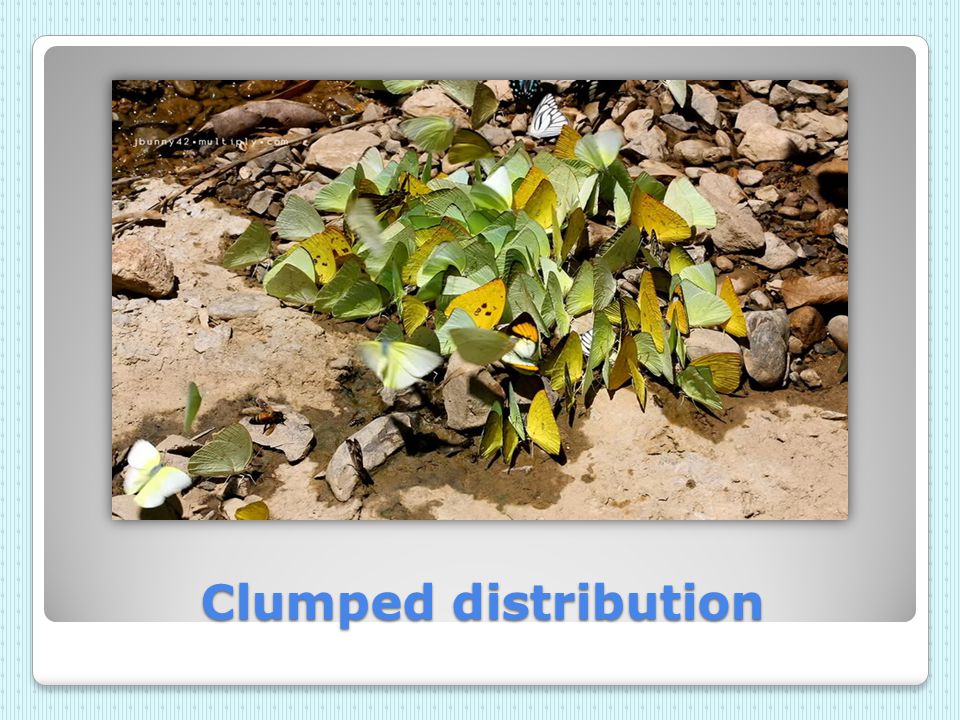The image is a detailed and colorful photograph depicting a natural scene, likely intended for educational purposes, perhaps a university course or botanical presentation. The setting is an outdoor environment featuring a small stream or water source flowing over rocks, creating a slightly wet area. Central to the image is a large number of butterflies, predominantly green and yellow in color, with some hints of white. These butterflies are clustered together in a clumped distribution on and around the rocks. The scene is accompanied by brown pebbles and dirt, enhancing the naturalistic feel. Below the main image, blue text reads "clumped distribution," and the entire composition is framed with a gray border, followed by a white border, and finally a light blue border, giving it a structured and layered appearance.